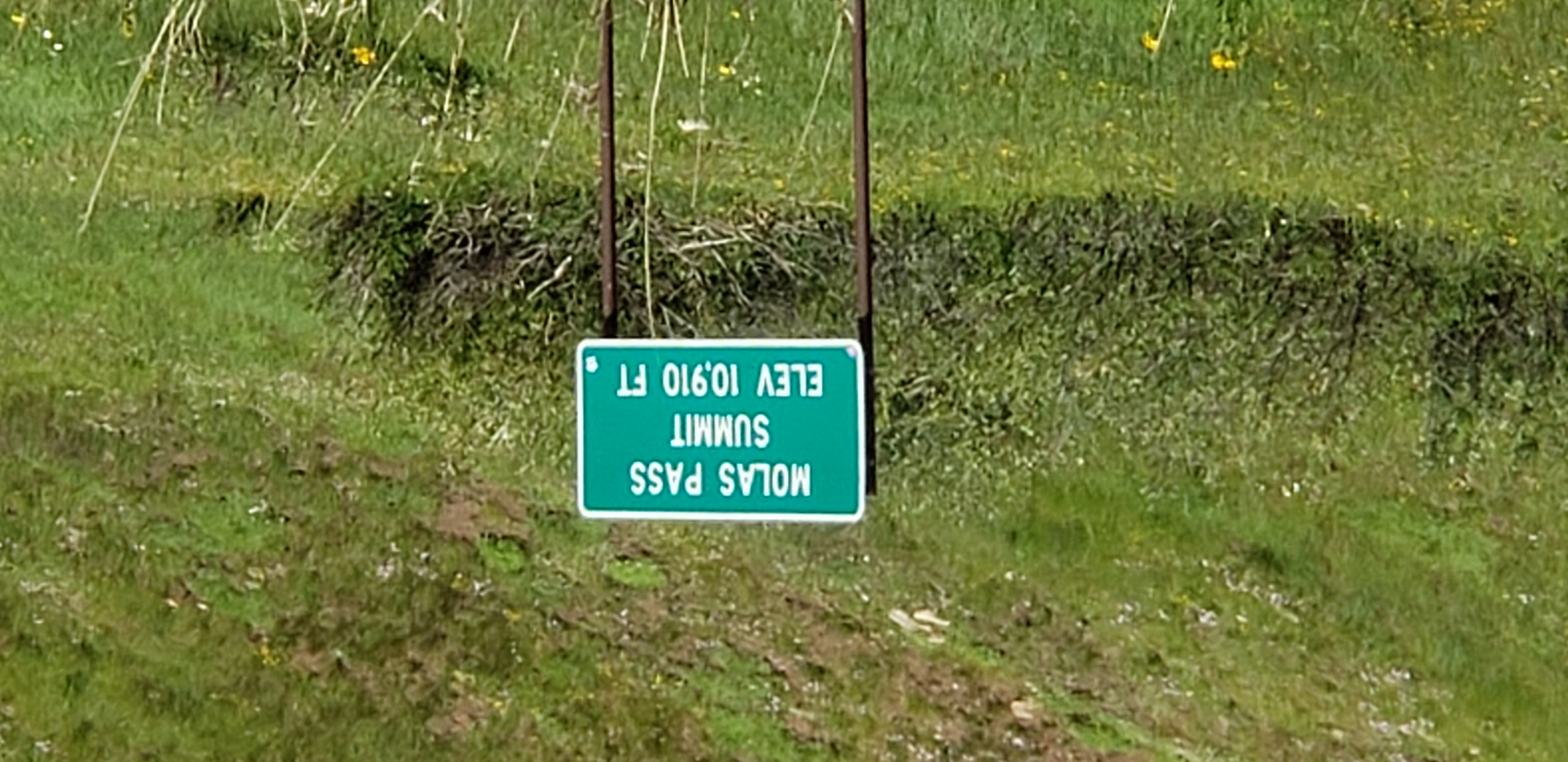The photograph depicts a sign along a hiking path or countryside trail, though it is shown upside down. When oriented correctly, the picture reveals a grassy hill area with some open dirt, low shrubs, and scattered rocks. It's likely summertime, as evidenced by the lush green grass and small yellow wildflowers starting to bloom. Centrally located, two metal posts support a green sign bordered with white reflective tape. The sign reads in white reflective text: "Molas Pass Summit, Elevation 10,910 feet."